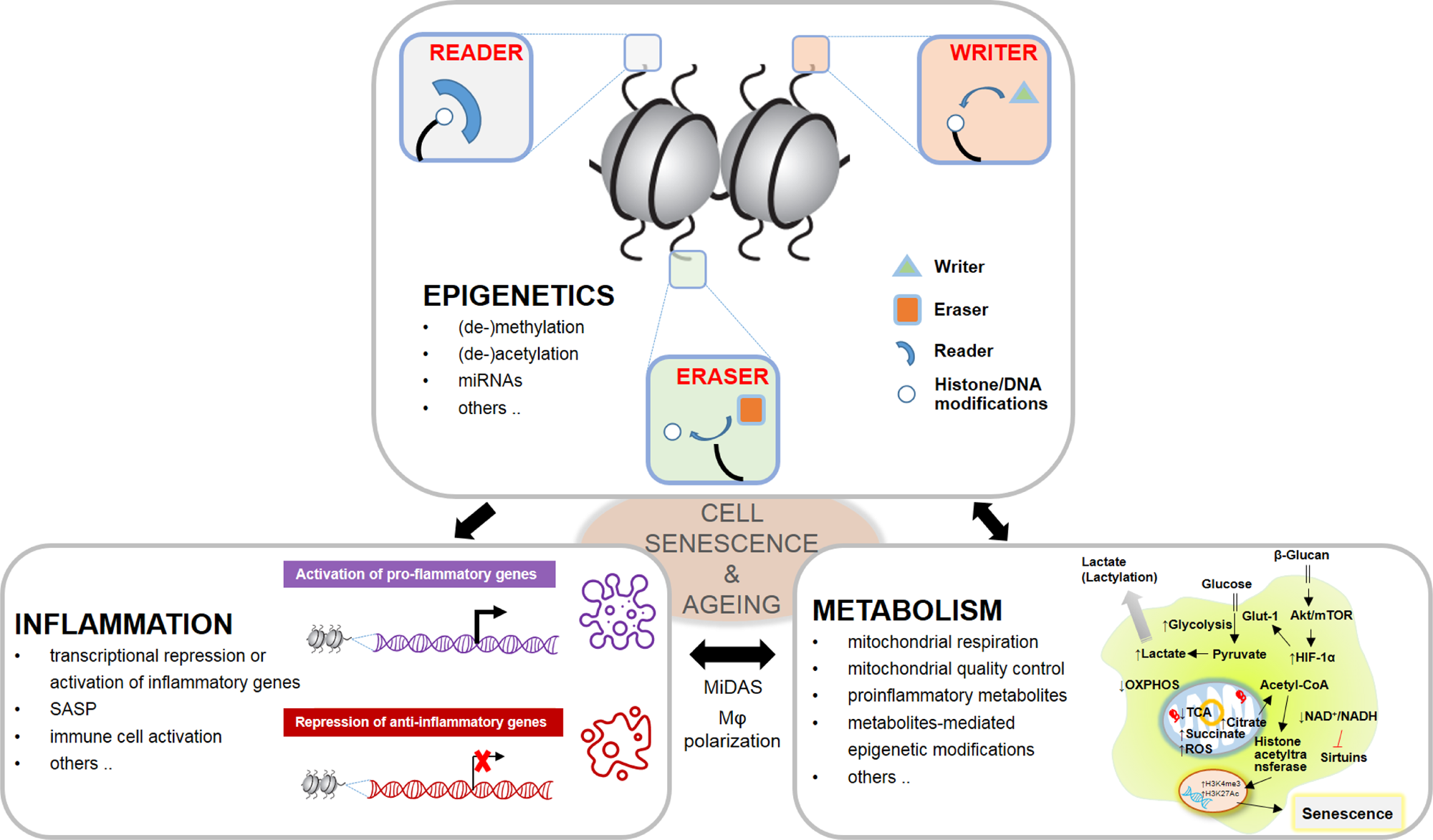The image is a detailed medical diagram presented as a flowchart with three main rectangular boxes forming a pyramid shape. At the center, there is a tan oval labeled "Cell Senescence and Aging." The top rectangle, which has a white background, gray borders, and rounded corners, is titled "Epigenetics." This box includes visual elements such as two round globe shapes with black lines around the gray shapes, and icons representing different epigenetic components: a teal triangle labeled "Writer," an orange square labeled "Eraser," and a curved blue shape labeled "Reader." The box also contains bullet points listing elements like "miRNAs and others."

Beneath this, two additional rectangles are positioned at the bottom left and right. The bottom left rectangle is labeled "Inflammation," featuring a bi-directional arrow, and includes a bulleted list under the title. To its right, the bottom right rectangle is labeled "Metabolism," also featuring a bulleted list. A black arrow points between these two bottom rectangles.

Overall, the diagram incorporates colors such as whites, grays, blacks, oranges, reds, purples, light beige, pale yellows, and green-yellow hues. The comprehensive labeling and use of color-coded symbols aim to represent the intricate processes related to cellular aging, epigenetics, inflammation, and metabolism.